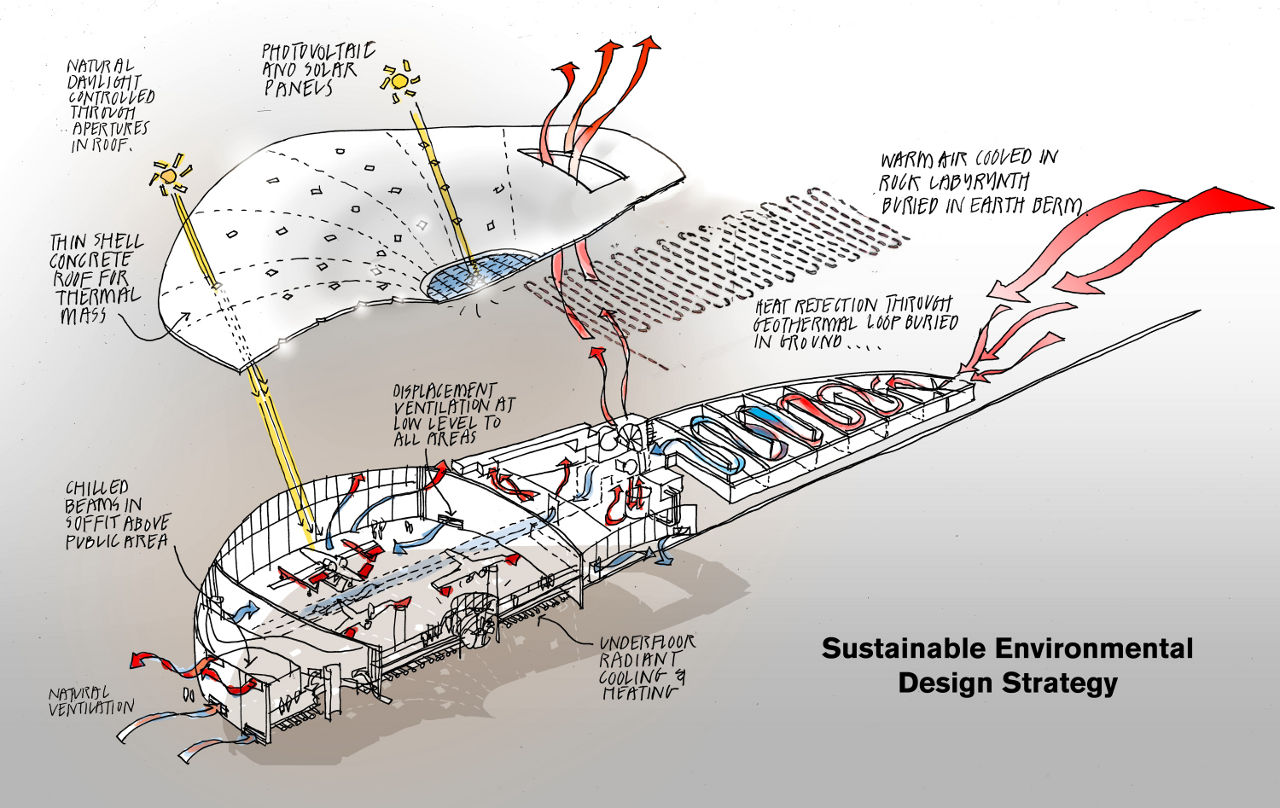This detailed drawing illustrates a comprehensive sustainable environmental design strategy for a building. The diagram prominently features an underfloor radiant cooling and heating system, with red arrows indicating the movement of warm air, which is converted into cool air through a series of processes. These include a rock labyrinth buried in the earth's surface for cooling and a geothermal loop for heat rejection. The design also incorporates natural ventilation, allowing the warm air to be expelled efficiently.

Photovoltaic and solar panels are strategically placed on the roof, which is composed of a thin shell concrete structure for thermal mass. This thermal mass helps to regulate the building's temperature. Natural daylight is harnessed and controlled through apertures in the roof, minimizing the need for artificial lighting and enhancing energy efficiency.

Additional features include chilled beams in the soffit above public areas and displacement ventilation at low levels throughout the building, ensuring air distribution is both effective and energy-efficient. The labeling throughout the diagram highlights these key elements, emphasizing the building's commitment to environmentally friendly and sustainable design practices.